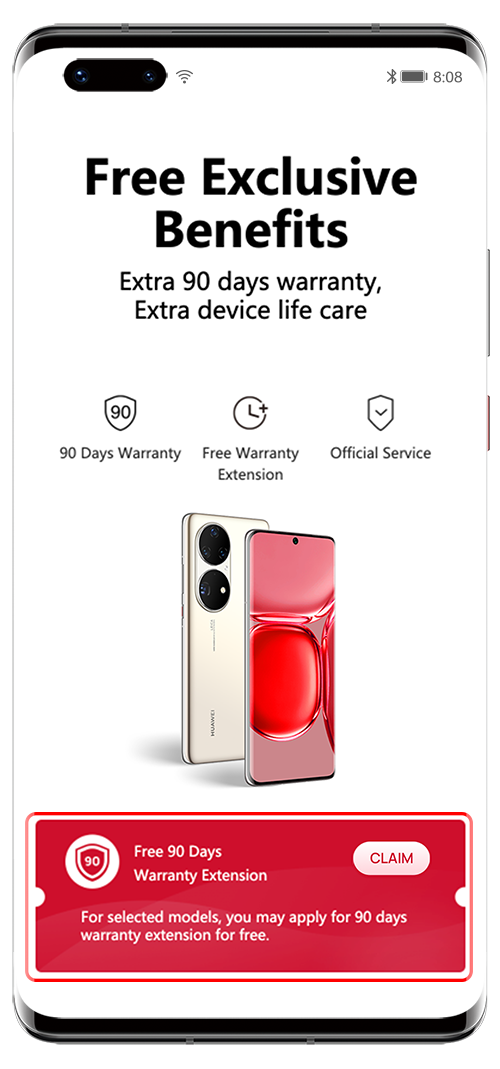Certainly! Here is the detailed and cleaned-up caption:

---

The image showcases a Samsung Galaxy mobile device, identifiable by the Android interface and the characteristic pill-shaped camera cutout in the upper left corner of the screen. The background of the screen is predominantly white, prominently featuring the text "Free Exclusive Benefits" in bold black letters at the top. Below this heading, the device displays several lines of text enumerating the benefits: "Extra 90 Days Warranty," "Extra Device Life Care," and "Free Warranty Extension." These benefits are further emphasized with additional text detailing, "Official Service."

Beneath this informational text, there is an image of a mobile device with a metallic gold or silver back and a striking pink and red colored display. Further down, a prominent red shield icon with the number "90" is visible, accompanied by the message, "Free 90 Days Warranty Extension for selected models. You may apply for a 90 days warranty extension for free." Completing the screen's messaging, there is a noticeable "Claim" button, inviting users to activate their warranty extension.

---

This caption provides a comprehensive description of the content and layout of the information presented on the device's screen.